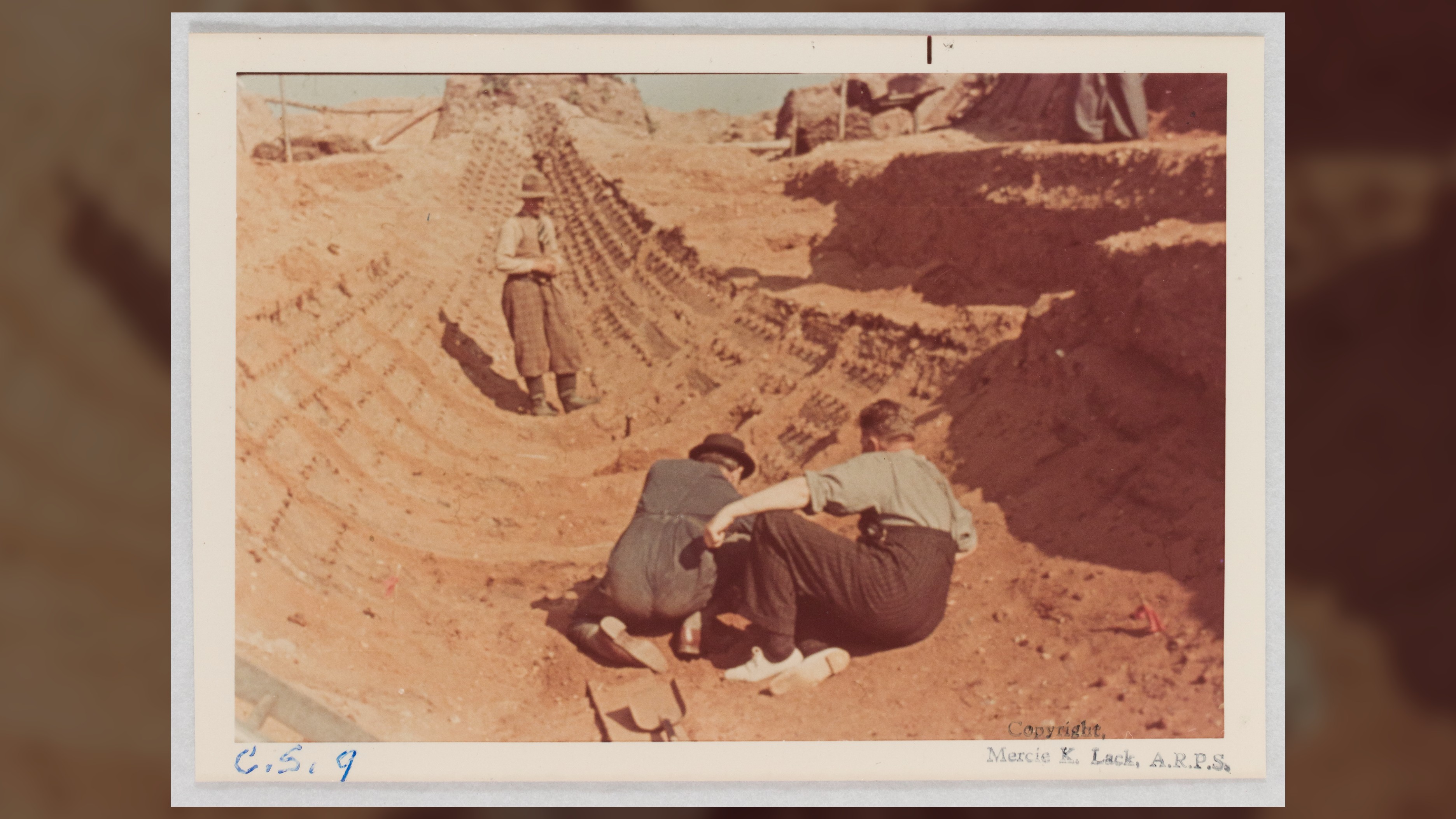The photograph features an outdoor scene, likely set in a desert or excavation site, with a reddish-brown dirt backdrop. The setting hints at an architectural or archaeological dig. The image is framed by a white border and bears the inscription "CS9" on the bottom left and "Marcy Elak AFPS" with a copyright mark on the bottom right.

In the foreground, two men are partially lying and bending over in a trench, intensely examining something on the ground. One of them is dressed entirely in black, while the other wears a white shirt paired with brown pants. Their backs are to the camera, adding an element of mystery to their work.

A third man, distinguished by a cowboy hat and baggy pants, stands behind them. He is dressed in a tan shirt and brown pants, and his presence suggests a supervisory role as he gazes towards the two men in the trench. The sun casts shadows, indicating a bright, sunny day, which further enhances the uniqueness of this excavation site amidst the arid, rocky roads.